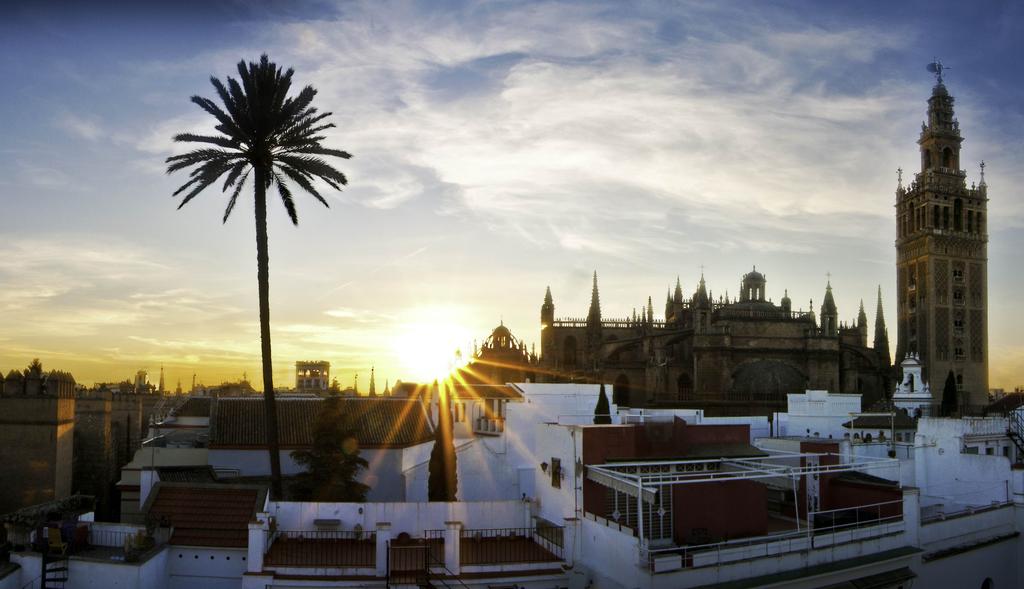In this photorealistic aerial photograph, a cityscape is captured during sunrise or sunset, illuminating the sky with a mixture of golden hues and wispy white clouds tinged with grayish blue. A prominently tall silhouette of a palm tree with a long, skinny trunk and a large, full canopy stands close to the left edge of the frame. The sun, slightly offset to the left of center, casts a bright, golden glow across the scene, giving a sense of warmth.

To the right, the city features a mix of buildings. A particularly noticeable tall structure with decorative turrets, reminiscent of a cathedral or castle, stands out among shorter, sandstone-colored and white buildings with flat surfaces and maroon roofs. The foreground reveals a few white buildings, their details shrouded in the shadow due to the bright sky. The architecture suggests a possible Middle Eastern location, though it's not explicitly clear. The overall composition is devoid of people, focusing solely on the serene, yet vibrant cityscape.